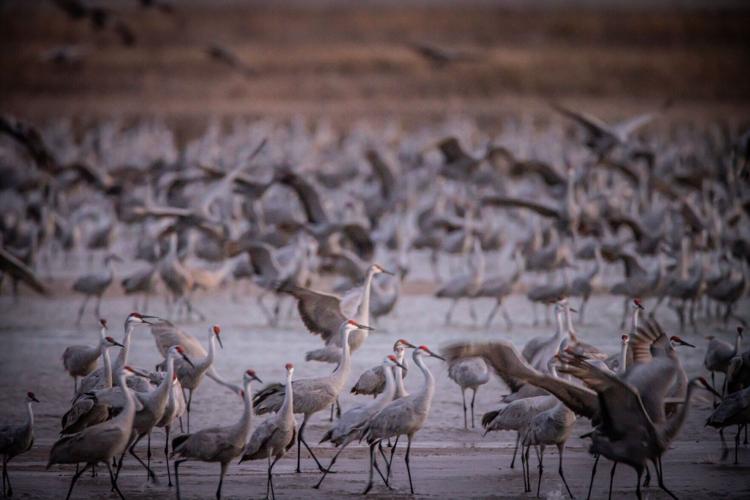The image captures a bustling scene of a large group of waterfowl birds in a shallow lake, teeming with activity. Predominantly whitish-gray with distinctive red markings around their eyes and on the tops of their heads, these birds resemble geese or cranes, although their exact species is uncertain. They possess long necks, blackish-brown or sharp black beaks, and slender legs. In the foreground, about 25 birds are clearly visible, while the background is populated with hundreds of others, creating a blurred effect. Many birds are wading through the water, plucking fish, with some standing or walking, and others mid-flight or taking off. The upper part of the image features a brownish landscape, possibly grass, adding depth to the scene. This captivating snapshot reveals the bustling life of these elegant birds in their natural habitat.